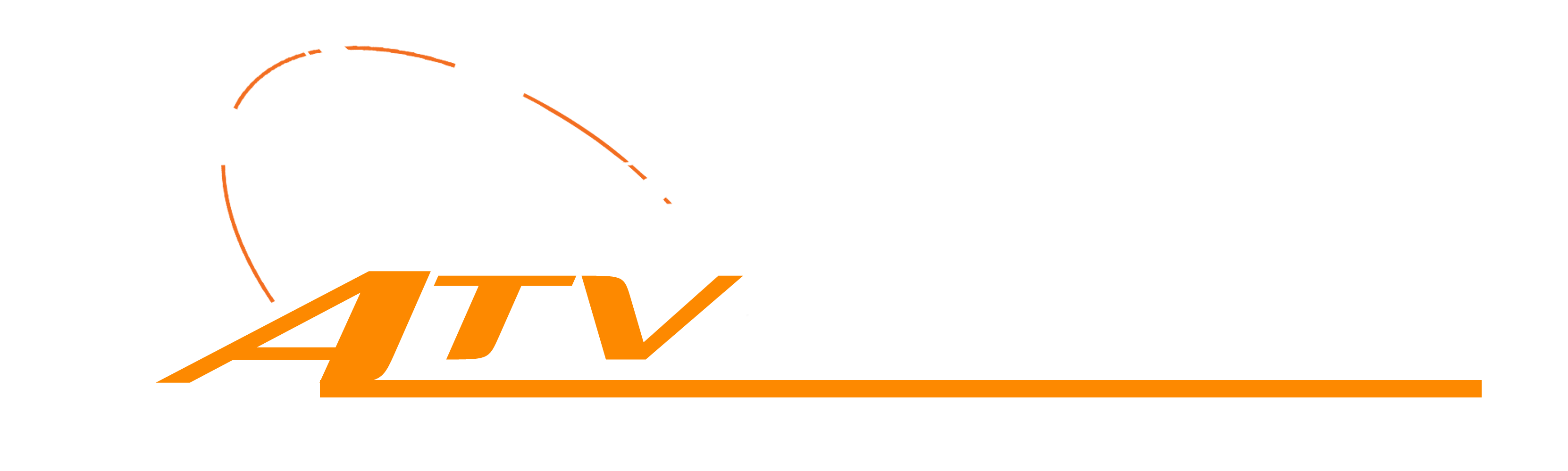The image is a minimalist logo set against a solid white background, featuring the bold, tangerine-orange letters "ATV" prominently. The letter "A" is angled, with its right side extending downwards to form a thick horizontal line that runs beneath "TV" and stretches across the image. Emerging from the left diagonal part of the "A" are four thin, dashed orange lines that create a semi-circular arc, curving over to end just above the opening of the "V". The design is clean and uncluttered, with no additional text, borders, colors, or imagery, emphasizing the simplicity and boldness of the logo.